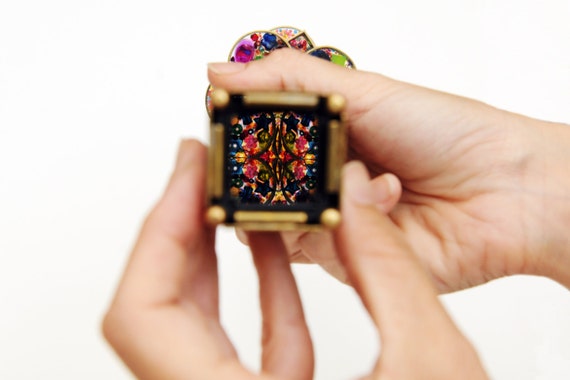In the image, two hands are prominently displayed holding a small, square object with blurred edges. One hand comes from the bottom gripping it with its fingers, while the other hand approaches from the right side, supporting the object from the back. The background is a plain white, adding to the overall blur and focus on the hands. 

The object itself has a metallic, gold square frame with rounded ball corners and a black inner outline. Within this frame lies a vivid, intricate design resembling a prismatic or kaleidoscopic image, divided into symmetrical quadrants. The central design showcases a multitude of colors including yellow, red, green, blue, dark blue, light blue, purple, and pink. This design appears to be abstract, with diamond-like lines and patterns that mirror each other both vertically and horizontally. Little black stars and floral elements add to its intricate detail. The overall impression is of a small, ornate, and colorful device being closely examined by the two hands.